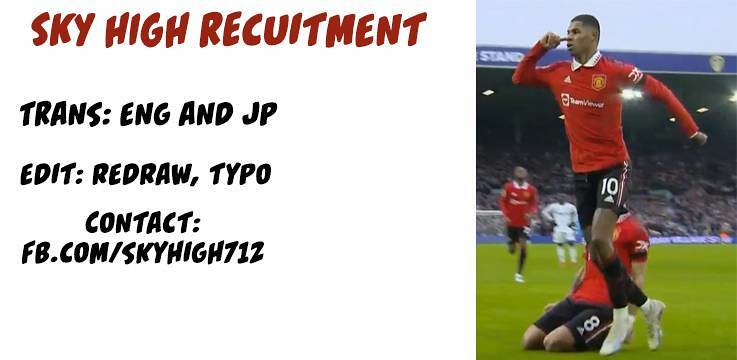The image captures an intense soccer match on a vibrant field. Players are donned in striking team uniforms: red jerseys with white collars and long sleeves, paired with black shorts. The central focus is on a dynamic player with the number 10 on his black shorts, caught mid-action with his feet off the ground. Behind him, a teammate with the number 8 on his shorts appears to be sliding or has fallen to the ground. A third player, also in red and black, rushes towards the action, while a referee in white stands further in the background. The stadium is teeming with spectators, adding to the charged atmosphere of the scene. Above the stands, there’s a prominent sign in red letters reading, "Sky High Recruitment." Below that, in black text, are the words "Trans: ENG, JP," followed by "Edit, Redraw, Typo." Further details for contact are provided at "FB.com/SkyHigh712."